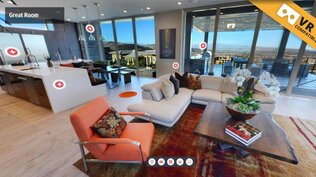The image depicts a virtual reality (VR) guest room with intricate detailing and vivid colors ranging from light orange, greens, yellows, blacks, whites, grays, reds, blues, beige, and tan. Positioned within a loft-style apartment, the scene captures a large open living space with a kitchen area on the left side. In the foreground, there's an orange accent chair paired with an L-shaped couch, centering around a glass coffee table. The far wall is lined with large window doors that overlook a valley and cityscape, enhancing the room's spacious feel. Numerous items are marked with red circles housing white plus signs, likely interactive points for the VR experience. These circles have white outlines and add a layer of interactivity to the room. In the top right corner, a yellow banner with black text prominently reads "VR," indicating the virtual reality interface. Additionally, a darker gray rectangle on the far left displays the text "great room," and there is a menu at the bottom of the screen, possibly for further navigation or options within the VR environment.